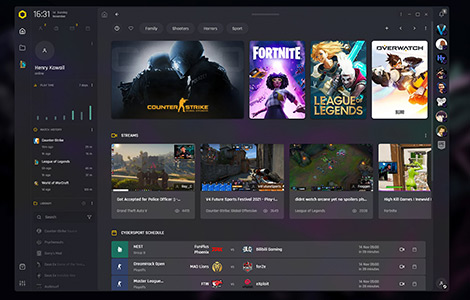This image depicts a webpage interface showcasing a variety of game options available for selection. At the top of the page, there are several icons including a yellow circle, a home button, and a file folder, along with a displayed time of 16:31. There is also a circular icon featuring a letter 'A' and a name in white text, suggesting a user profile or account indicator. 

Below this, there are several green-colored bars, possibly representing a loading or progress indicator. The webpage categorizes games into different tags such as "Family," "Shooters," and "Sports." 

The first game listed is "Counter-Strike," highlighted in yellow text, featuring an image of two characters in uniforms and helmets, suggesting a war or tactical shooter game. 

Following that, there is a prominent "Fortnite" poster displaying a character with glasses set against a bright purple background with "Fortnite" written in bold white text. 

Next is "League of Legends," featuring a blonde character in a uniform with what appears to be an evil character beside them. 

"Overwatch" is also listed, showcasing a character that resembles a flying superhero in a costume.

The page predominantly features a gray background adorned with various images and game artwork, accompanied by numerous icons and settings options for user navigation and customization.